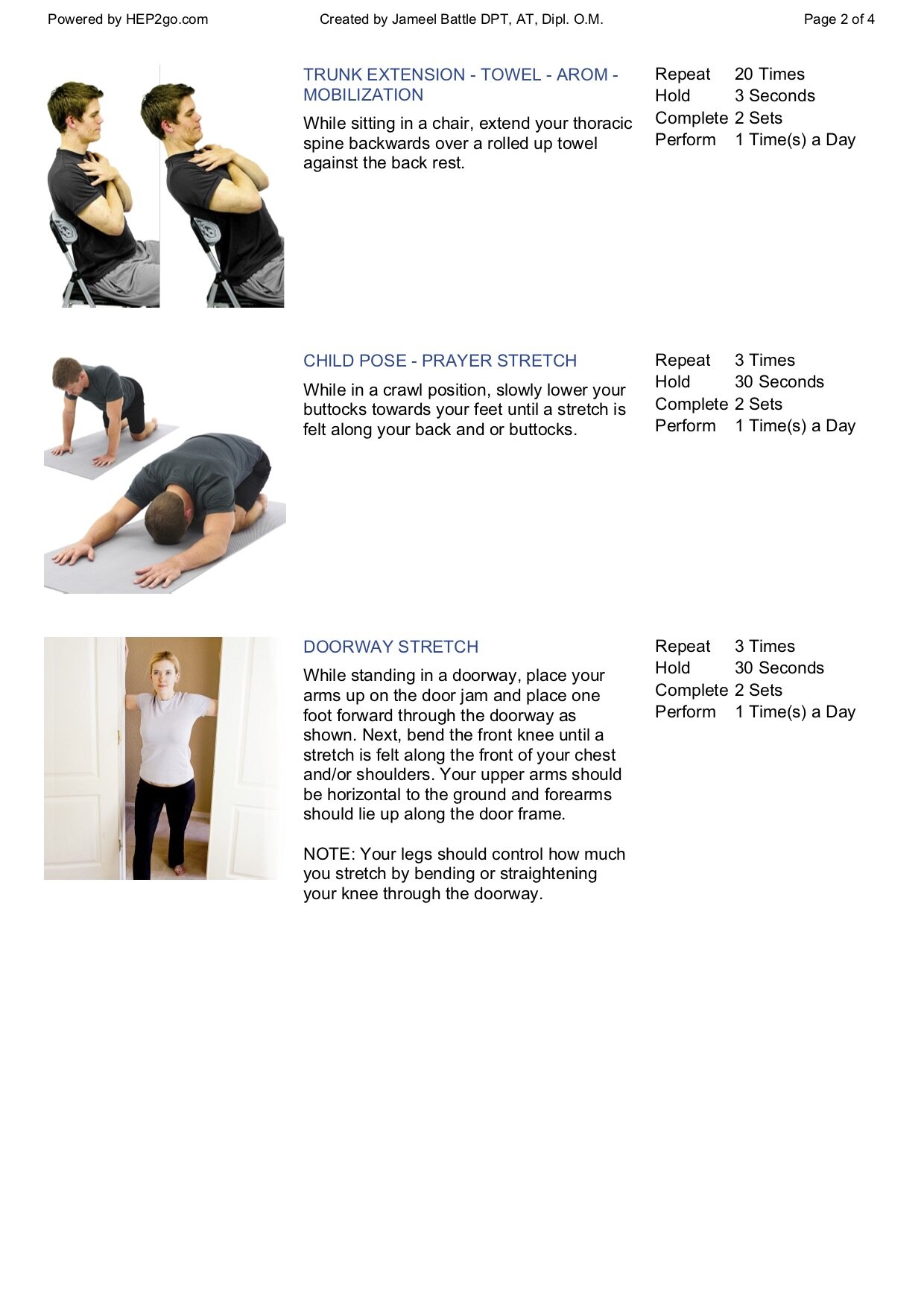The image, powered by HEP2Go.com and created by Jameel Batty, DPT-AT-DPOM, displays detailed instructions for performing three different stretches. At the top left corner, it's labeled as page 2 of 4. The first stretch is the Trunk Extension with Towel Arm Mobilization. It shows a person sitting in a chair with their hands crossed over their chest, leaning back against a rolled-up towel positioned against the backrest to extend the thoracic spine. The instructions state to repeat this movement 20 times, hold each extension for 3 seconds, complete 2 sets, and perform the exercise once a day. The second stretch is the Child Pose or Prayer Stretch. The depiction includes a person starting on all fours, then leaning back with their buttocks moving toward their feet to stretch the back and buttocks. This pose should be repeated 3 times, held for 30 seconds each time, completed in 2 sets, and performed daily. The final exercise is a Doorway Stretch, illustrated with a woman standing in a doorway with her arms resting on either side of the door frame. She steps one foot forward and bends the front knee to create a stretch along the chest and shoulders, while the arms are kept horizontal to the ground and aligned with the door jamb. This stretch is to be repeated 3 times, held for 30 seconds, completed in 2 sets, and performed once a day.